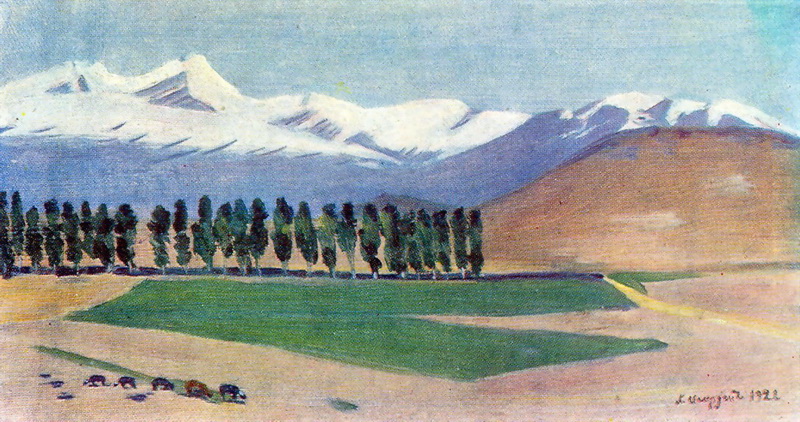The painting portrays an idyllic landscape in a stunning blend of colors and details. The sky, effortlessly light blue without a single cloud, spans the top of the painting, setting a serene mood. Below this tranquil sky lies a majestic mountain range, its peaks capped with pristine white snow and dark gray bare rock. Nestled at the foot of these mountains is a large brown hill, adding a contrasting earthy tone to the composition.

In the mid-ground, a winding road or river seamlessly traverses the scene from left to right, flanked by slender, green-leaved trees that stand like sentinels along its path. The foreground is dominated by a vast field, interspersed with various green patches and brown soil. To the right, a distinctive yellow road cuts through the landscape, adding depth and direction to the painting.

On the bottom left, a cluster of cows, their heads bowed as they graze, brings life and movement to the scene. A signature adorned with the numbers "1922" in black ink graces the bottom right corner, marking the artist's completion of this landscape masterpiece. The meticulous details and harmonious color palette evoke a sense of peace and natural beauty, capturing the essence of a timeless countryside.